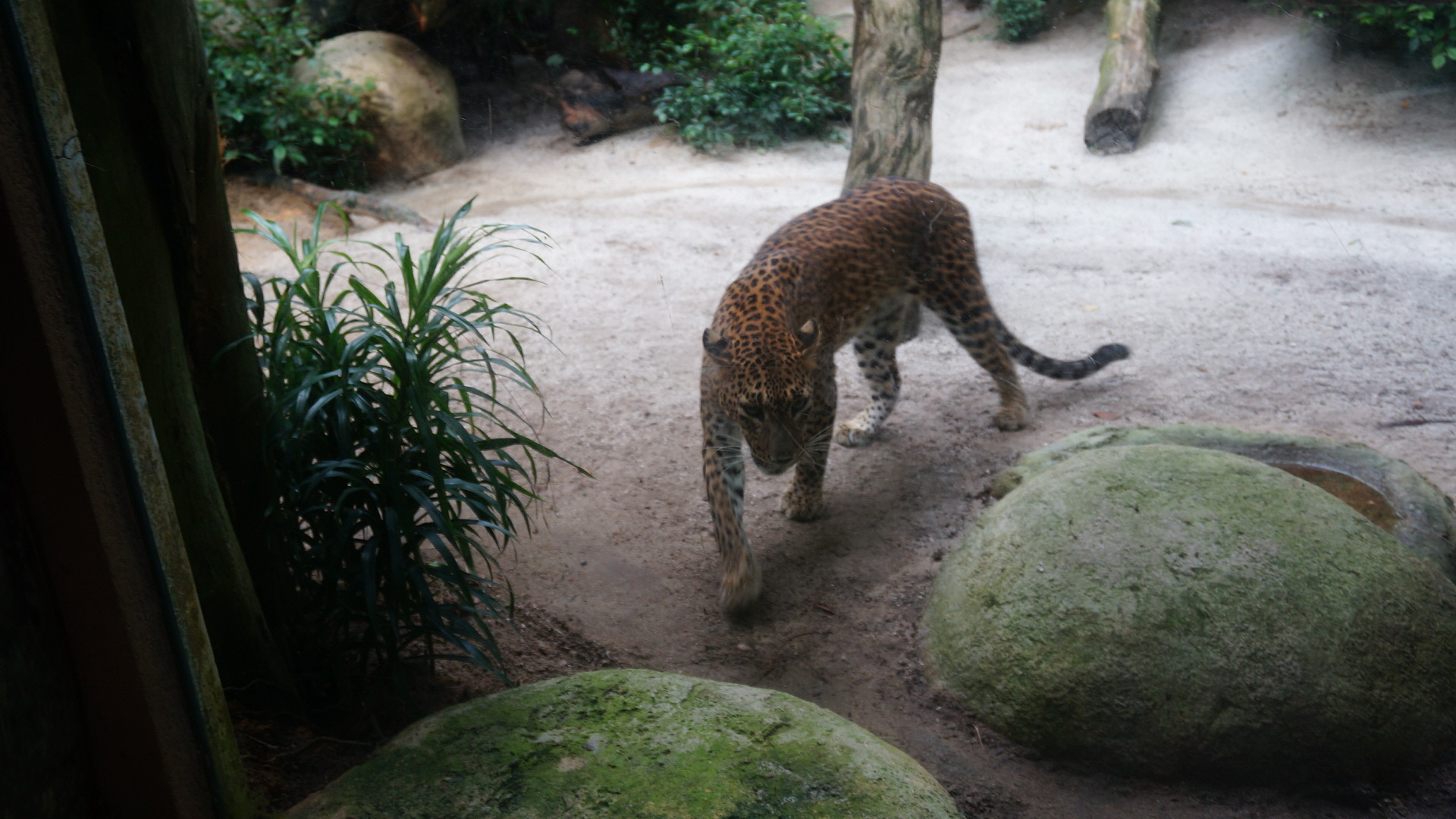This photograph captures a vibrant scene of a cheetah in a well-lit zoo enclosure during the daytime. The cheetah, adorned with a striking coat of orange fur covered in black spots and a tail featuring white and black stripes, is confidently walking towards the camera over sandy terrain. In the foreground, two large, moss-covered boulders complement the naturalistic setting, while additional boulders can be seen towards the back left corner. The enclosure is rich with greenery, including bushes, shrubs, and a sprawling tree on the left that provides ample shade. Behind the cheetah, there are more trees and some fallen logs, adding to the authenticity of the habitat. A partially visible structure resembling a wall borders the left side of the picture, hinting at the enclosure's boundaries while blending seamlessly into the environment. The overall composition suggests a serene outdoor environment, meticulously designed to mimic the cheetah's natural habitat.